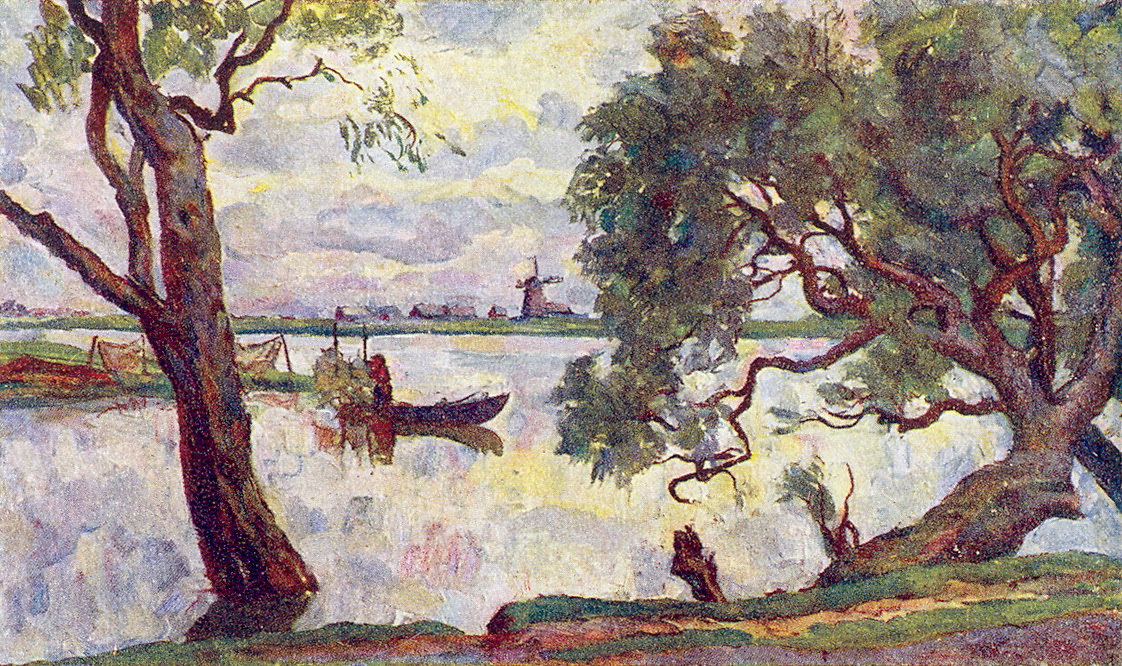The painting is a horizontal rectangular depiction of a tranquil lakeside scene reminiscent of the era of the Dutch masters. In the foreground, green grass edges the lake, leading to two unusually shaped trees growing directly from the water, their branches stretching in all directions. Nestled between these trees is a small wooden rowboat, occupied by a person. Along the shore, a few more boats are tied, and to the left, lean-to tents can be seen. The water, painted in soft pastel shades, reflects the sky’s serene palette of blues, yellows, and hints of pink. The distant background features several cottages and a prominent windmill, towering over the village houses. The overall scene, with its detailed greenery, rustic boats, and mirrored sky, creates a picturesque and peaceful atmosphere, highlighting the beauty of the natural landscape.